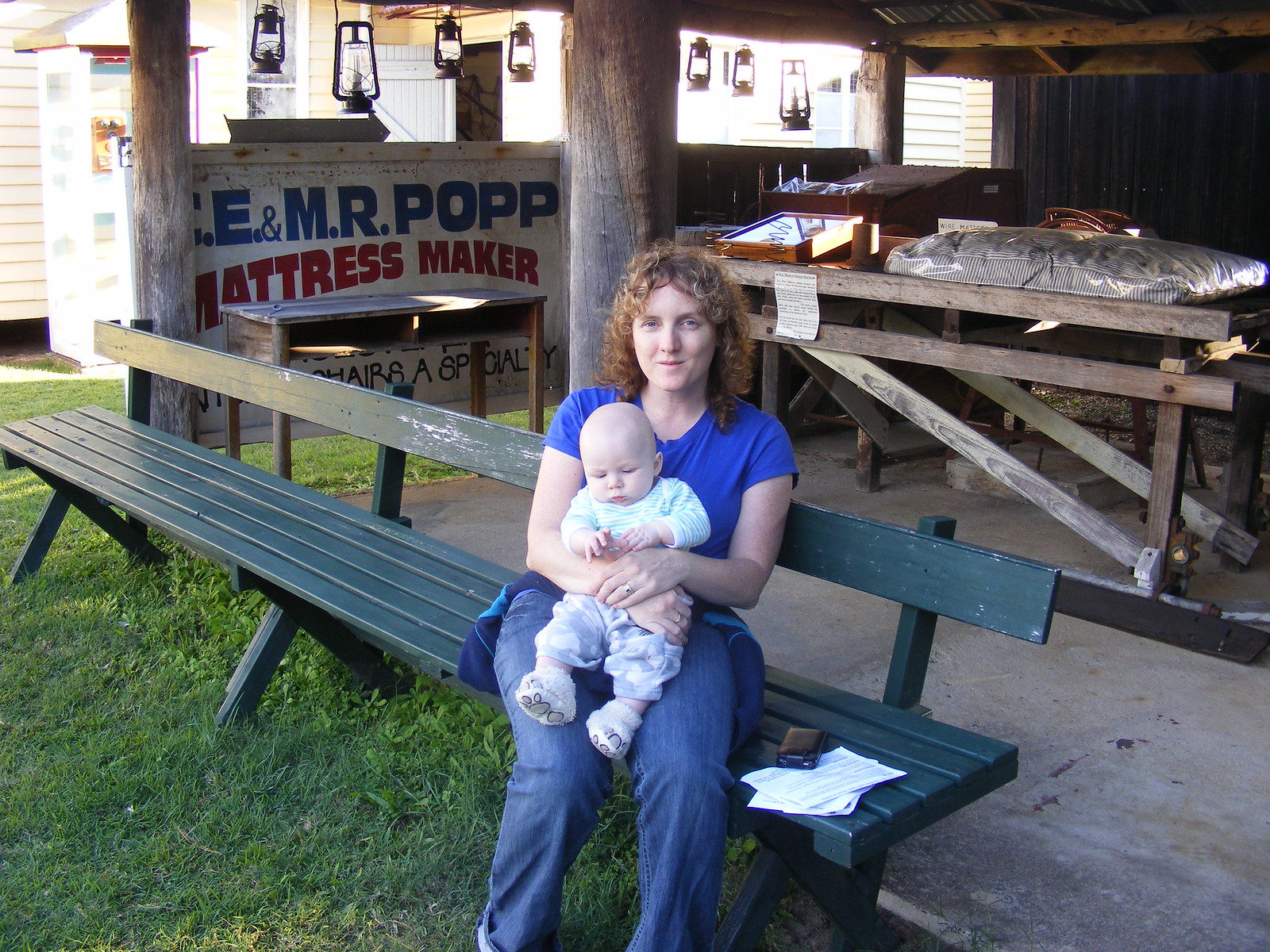In an outdoor photograph, a woman with curly, light brown hair sits on a long green wooden bench, which stretches diagonally from the lower right to the upper center of the image. Dressed in a blue short-sleeved shirt, blue jeans, and with a blue sweater tied around her waist, she looks directly at the camera while holding a baby on her lap. The baby, dressed in a light blue and white striped jumper, blue pants with cloud patterns, and booties designed to look like polar bear paws, gazes downward. 

Behind them is a white building that resembles a barn, adorned with wooden tables and hanging old oil lanterns, suggesting a rustic setting. A notable sign in the background reads "C.E. & M.R. POP Mattress Maker" in blue and red letters, positioned above the central portion of the bench. The ground beneath the bench is grass, transitioning to a concrete floor under the table behind her, which holds various items, possibly including a transparent container. The scene captures a moment of serene interaction amidst a quaint, rustic backdrop.